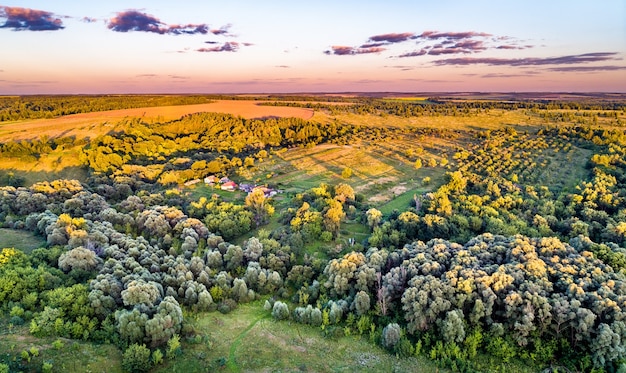This aerial image showcases a vast and vibrant landscape dominated by a sprawling field of trees and greenery transitioning into autumnal hues. The foreground features numerous trees, some still green while others are turning a striking yellow, indicative of the fall season. There are neatly planted rows, possibly of trees or large flowers, with clear spaces between them, adding to the orderly beauty of the scene. At the center of the image, a large open field stands out, uniformly blanketed in yellow, creating a vivid contrast.

In the distance, a flat mountain covered with a yellowish hue extends into the horizon, subtly blending with the rest of the landscape. The ground perhaps owes its yellow tint to the sandy clay dirt predominant in the area. The expansive sky adds to the enchanting ambiance with its spectrum of colors - shades of pink and purple merging into a light blue, suggesting the tranquil moments of either dawn or dusk. Puffy clouds reflecting pink hues drift across the sky, casting soft shadows below. The horizon is tinged with cream and blue, completing the picturesque and serene setting devoid of any people or animals. Overall, the scene feels almost surreal yet exudes a heartwarming, pleasant mood.